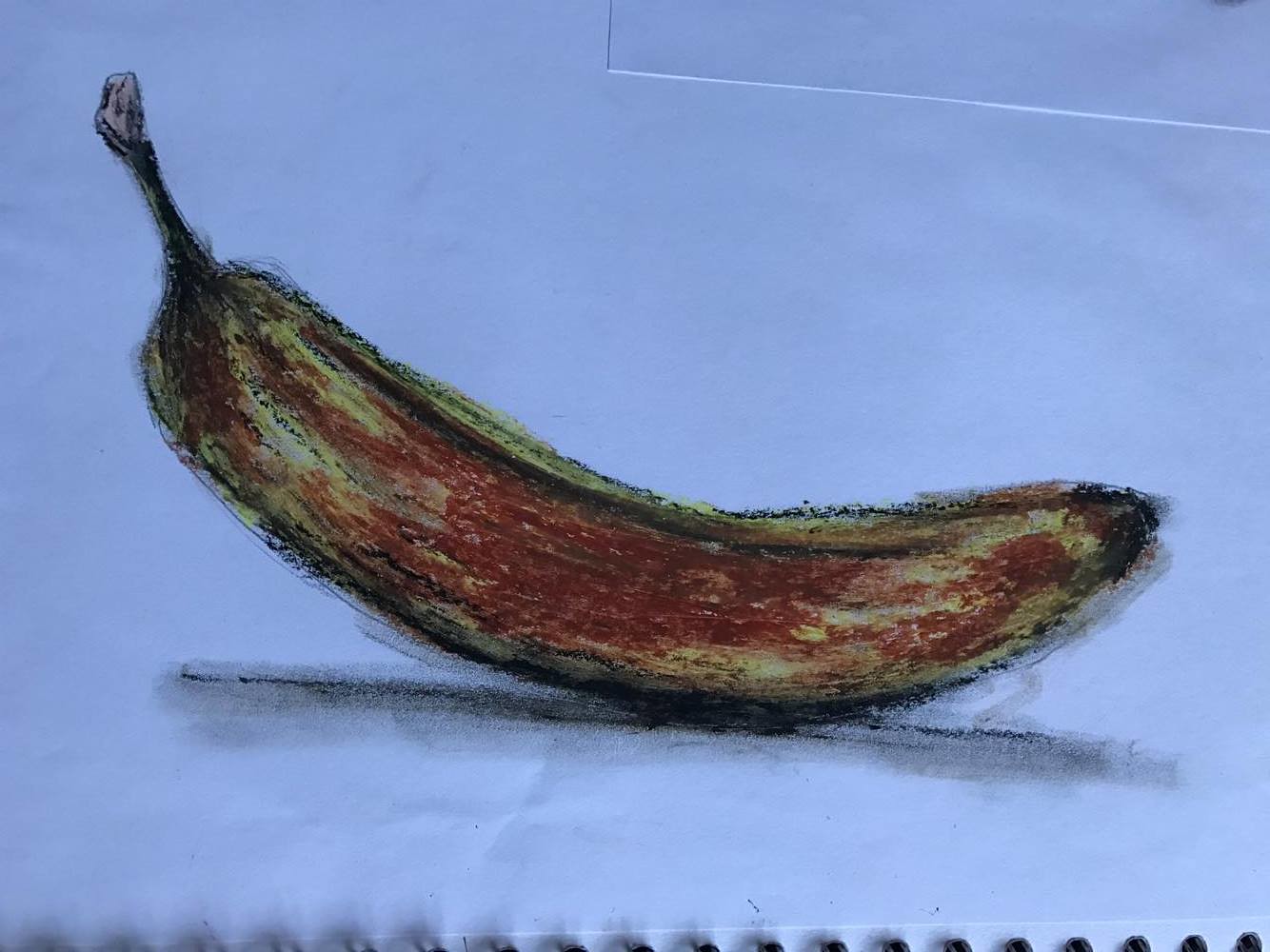This illustration features a meticulously detailed drawing of a banana, set against a pristine white spiral sketchbook page. Central to the image, the large banana is prominently outlined in bold black ink, capturing the eye. The banana exhibits a fascinating color scheme: while primarily yellow, the middle section is intriguingly shaded in red, with additional red spots adorning the top right end and near the stem. The stem, oriented to the top left, directs the banana's curved form upward. The lower portion of the banana, pointing right, rests centrally on an implied surface, with shadowing achieved through charcoal pencil, adding depth. Visible spirals from the notebook frame the bottom of the composition, while a rectangular cut-out in the top right corner of the page adds an interesting, irregular detail.